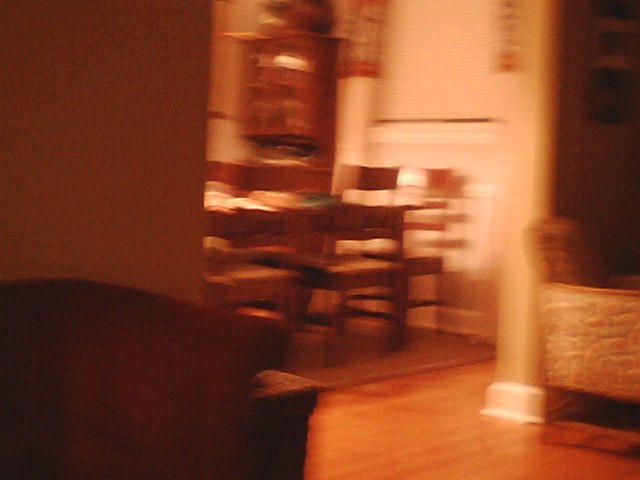This blurry image appears to be taken indoors, possibly inside a house or an apartment with a homely atmosphere. The flooring is hardwood with a high polish finish, displaying a medium brown tone, though an unusual glow affects the image's overall color. Despite the blur, wooden chairs typical of a dining room set can be discerned, arranged around a faintly visible table surface. The table’s details are obscured, making it unclear if there are objects on it or just blurry reflections. 

In the background, a white window shade is drawn down within a white window frame, framed by light-colored walls and possibly accented by red curtains that are pulled open. The image also suggests the presence of wood cabinetry within the room. The scene is viewed from a darker adjacent room through an open archway. This adjoining space appears to be a living area, with a comfortable-looking chair and another piece of furniture discernible in the shadows.